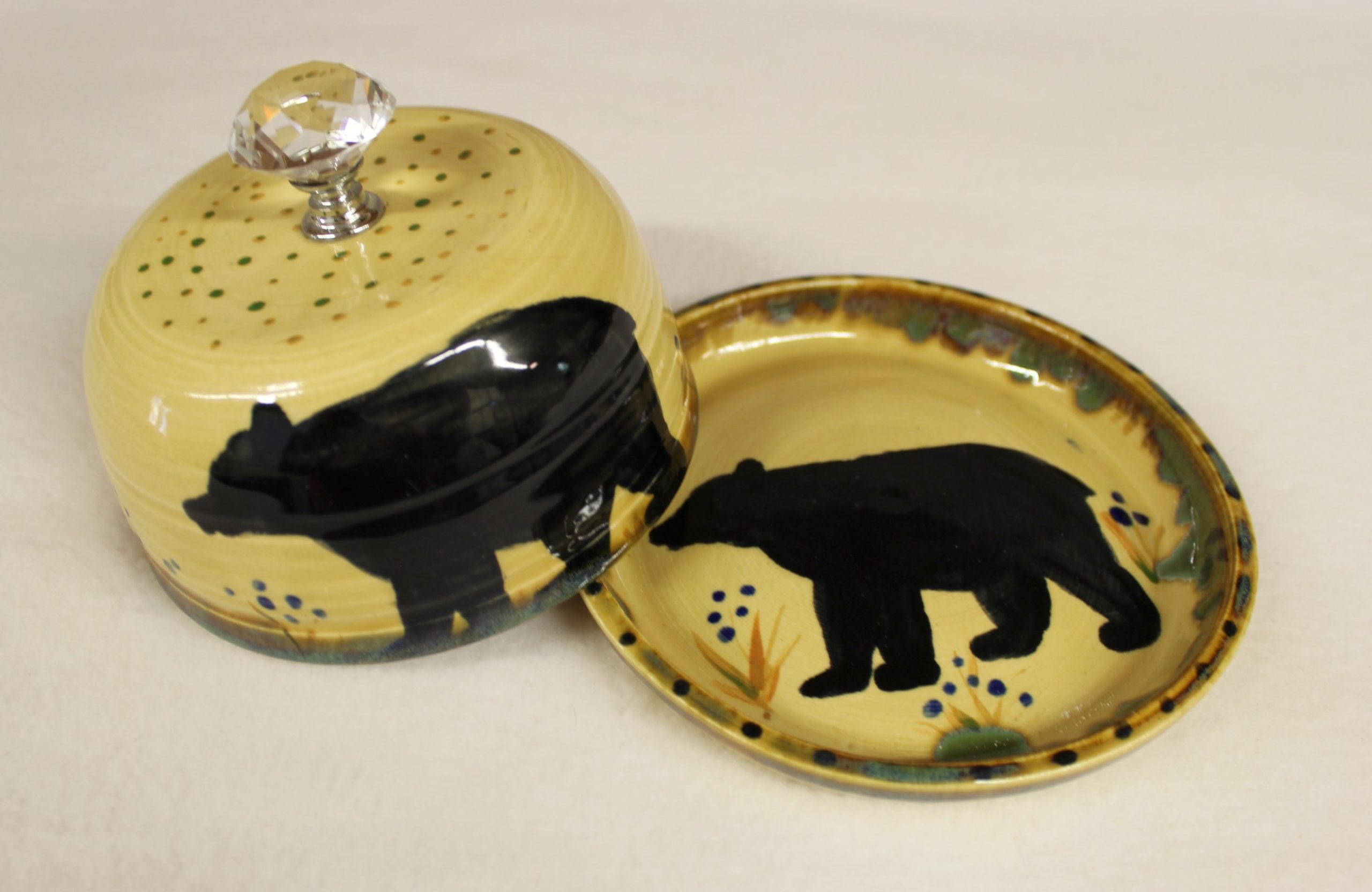In this detailed indoor photograph, a round, glazed pottery plate accompanied by its dome-shaped cloche cover is displayed on a light purple surface that fills the background. Both the plate and the cover share a main color of yellowish tan with light brown undertones. Positioned towards the lower right of the rectangular image, the plate features intricate designs: a black bear painted in the center facing left, framed by yellowish and green plant motifs with blue dots symbolizing rocks and stones around them. The outer rim of the plate is adorned with blue polka dots. Resting partially on the plate and partially on the surface to the left, the cloche mirror's the plate's artistry—it also boasts a black bear surrounded by blue and brown polka dots on its domed top. Completing the ornate lid is a clear, crystal handle with a silver base, contributing to the elegance and coherence of the entire set.